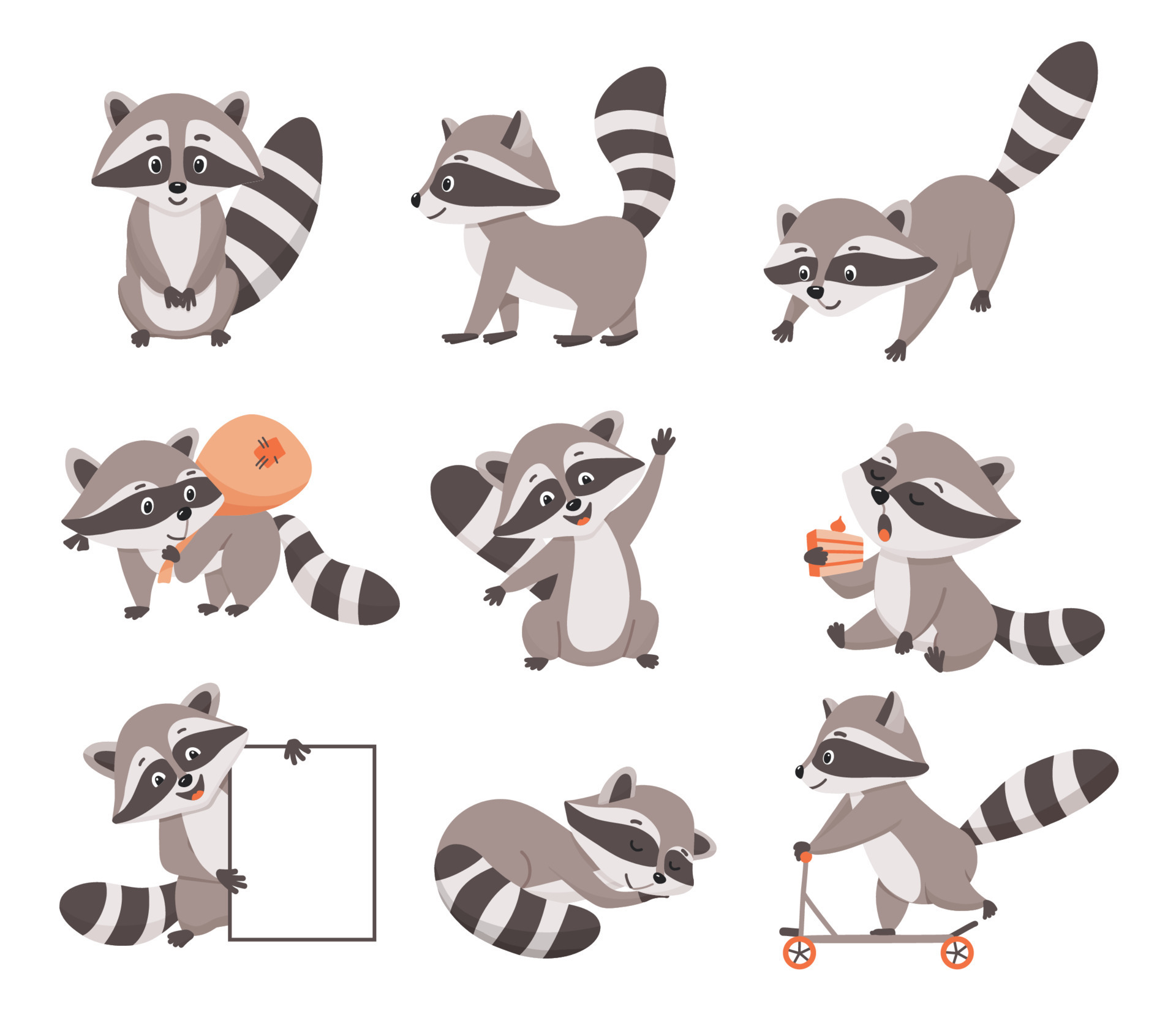This image showcases a grid of nine computer-generated cartoon raccoons in a variety of playful poses and activities, arranged in three rows and three columns. Each raccoon is predominantly gray with distinctive white and black facial markings, a gray-black striped tail, and perked-up ears.

In the first row:
1. The top-left raccoon is standing upright, facing forward with its front paws clasped together, resembling a child standing with hands together.
2. The middle raccoon is in profile, walking to the left with its tail raised.
3. The raccoon on the right is crouching playfully on all fours, with one paw extended forward.

In the second row:
1. The left-most raccoon stands facing right, carrying an orange sack and wearing a bandana over its eyes, hinting at a mischievous heist.
2. The center raccoon stands with its arms outstretched, one up and one down, as if greeting or offering a hug with a smile.
3. On the right, the raccoon sits down, mouth open, holding a piece of peach-colored birthday cake, possibly about to blow out the flame on top.

In the third row:
1. The raccoon on the left is smiling and holding a white rectangular board or mirror.
2. In the middle, another raccoon is curled up, seemingly asleep.
3. The raccoon on the right is riding a scooter, happily moving forward with a joyful expression.

Every raccoon is depicted with careful attention to their endearing characteristics, from their detailed coats to their expressive faces, making this collection a delightful visual treat.